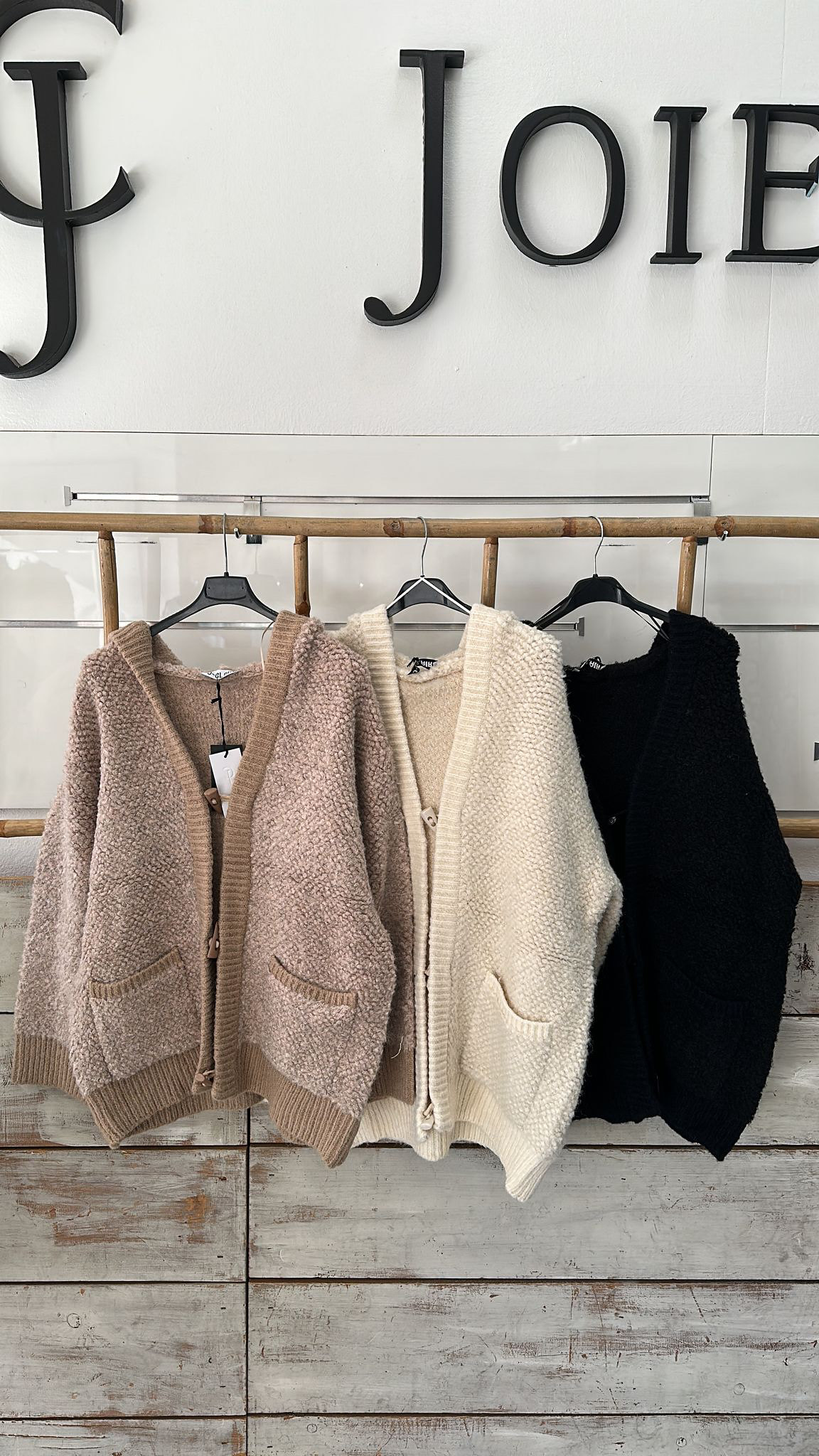The image is a high-end, color photograph, likely from a professional source such as a website or magazine advertisement. It features a store called Joie, with the store's name "Joie" (J-O-I-E) prominently displayed on a white wall. To the left of the name is a stylish logo consisting of a black C overlapping a black J, with the J intersecting the lower arc of the C. The lower portion of the wall has a distressed, reclaimed barn wood appearance, giving it a rustic yet sophisticated feel.

In front of the wall is a wooden rack, possibly bamboo, held in place by metal rods. Hanging on this rack are three sweaters, all of the same design but in different colors. The leftmost sweater is a dusty rose or light brown with a slightly darker trim around the opening and bottom, featuring patch pockets, a ribbed collar, and a zip front. The middle sweater is a cream or light beige color, and the one on the right is entirely black. Each sweater hangs from a black plastic hanger with a metal hook, and they all have visible labels inside. The overall setting conveys a muted, natural, and expensive ambiance.